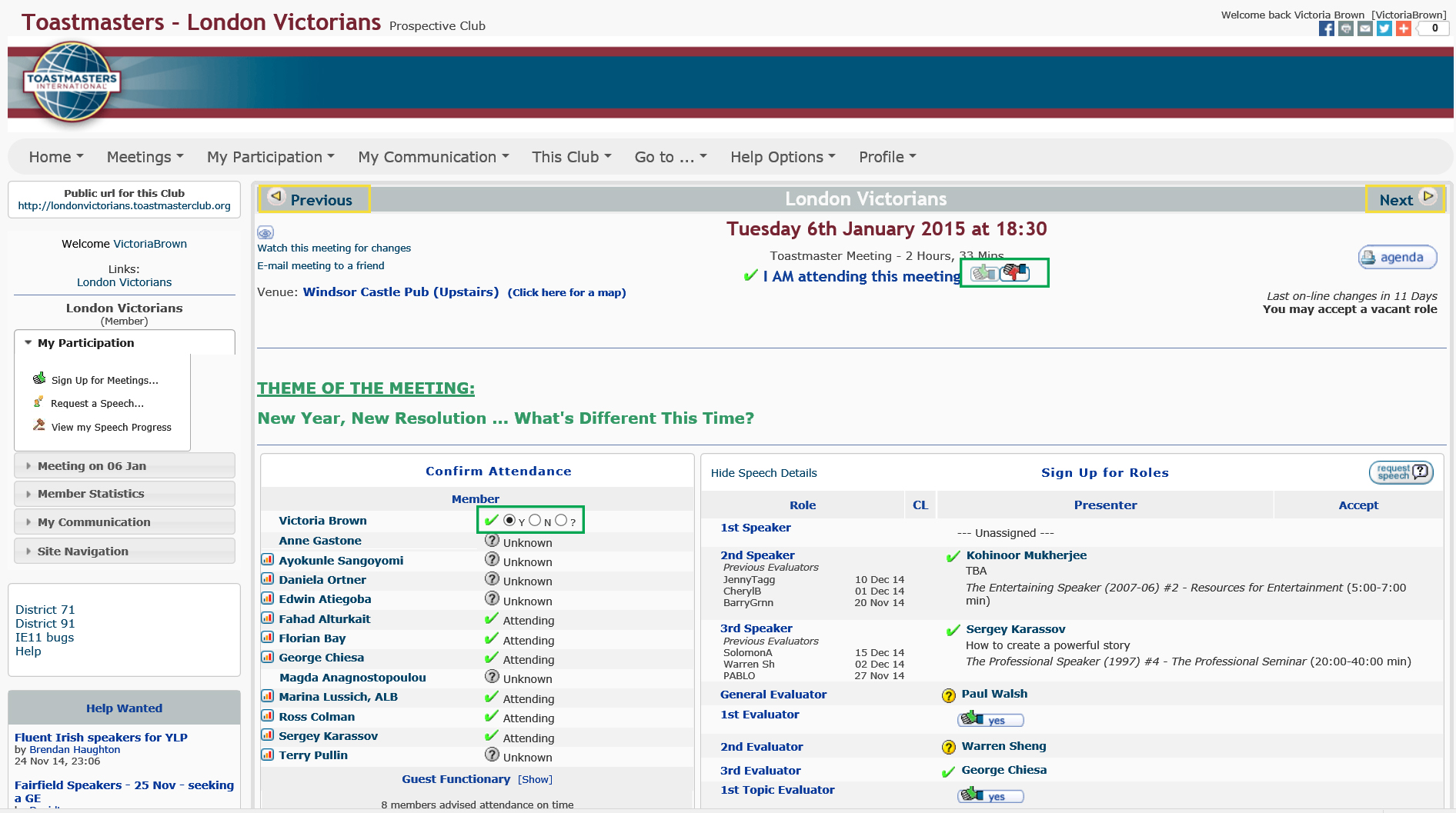Toastmasters International - London Victorians Club Meeting.

Welcome back, Victoria Brown!

Join us for an engaging session on Tuesday, January 6, 2015, at 6:30 PM. The meeting will be held at the Windsor Castle, upstairs venue. This Toastmasters meeting, home to Tez's participation and communication improvement, will last for 2 hours and 30 minutes. 

The theme of the evening is "New Resolutions: What's Different This Time?" led by our esteemed leader. 

Prospective members and guests are encouraged to attend and see the dynamic presentations and speeches. For more details, visit our public URL at http://londonvictorians.toastmasterclub.org. 

Stay tuned for updates on future meetings, and don't forget to confirm your attendance. Feel free to share this invitation with friends.